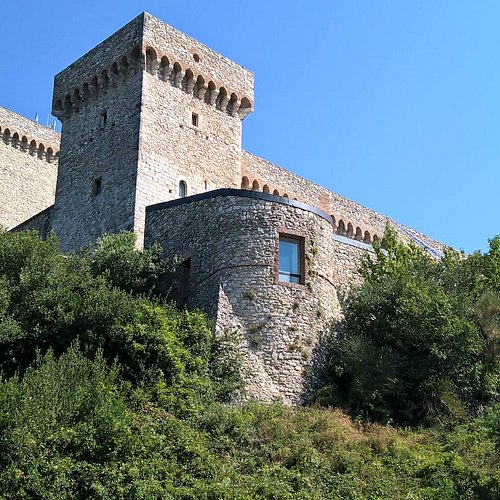A stunning, low-angle photograph captures a majestic stone castle nestled atop a verdant hill against a bright blue sky. The castle, composed of light brown stones, features an intricate blend of medieval architecture with modern elements indicating recent restoration. In the foreground, lush green trees and grasses frame the structure. A prominent rectangular tower on the left side boasts a distinctive row of rectangular cut-outs with rounded tops near its peak, flanked by two small windows on the front and left sides. Adjacent to this tower, a shorter, round tower features a large rectangular window with a metal border at the top. The upper section of the image reveals a wider, horizontal wall extending behind the towers, leading to additional parts of the castle adorned with numerous arched windows or doorways. The immaculate condition and modern amenities suggest that this historic structure may have been repurposed, possibly as a residence or a hotel, seamlessly blending its ancient charm with contemporary comforts.